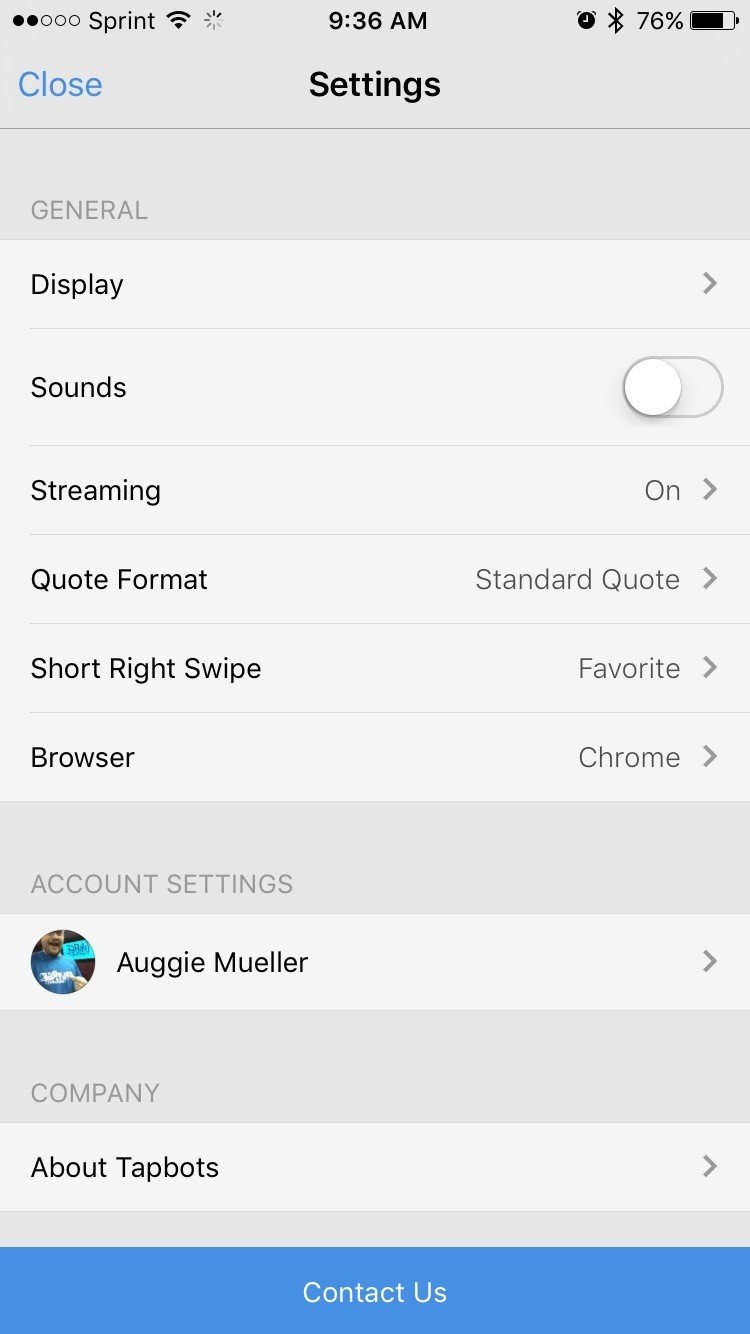A detailed profile image features an individual wearing a blue shirt layered with a white shirt that has a blue logo. The person has a well-groomed beard and stands against a black square backdrop. The background behind the black square is blue with white writing. The screen displays various UI elements: "Sprint" carrier information, time "9:36 AM", and a "76% battery" indicator. Connectivity indicators show active Bluetooth, Wi-Fi, and Sprint service. Other visible toggles and icons include general settings, a browser shortcut for Chrome, account settings, and buttons labeled with functions such as "Favorite," "Alarm," and "Loading."